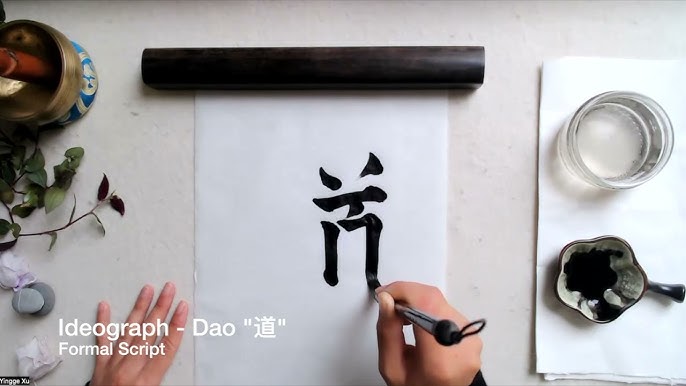The image captures an overhead view of a person engaged in the meticulous process of Chinese calligraphy. The bright white paper, possibly a scroll, is the canvas under the hand holding a brush, poised in mid-action, crafting a single, elegant character in formal script with rich black ink. To the right of their hand lies a small inkwell with black ink and a clear glass of water, both resting on what appears to be a white tablecloth atop a marble table. On the left side, there's a cup containing various pens. Overlapping the person's left hand is white text that reads "ideograph-dao," accompanied by Chinese or Japanese characters, along with the notation "formal script," emphasizing the calligraphic and formal nature of the work. The overall scene conveys a sense of traditional artistry and precision.